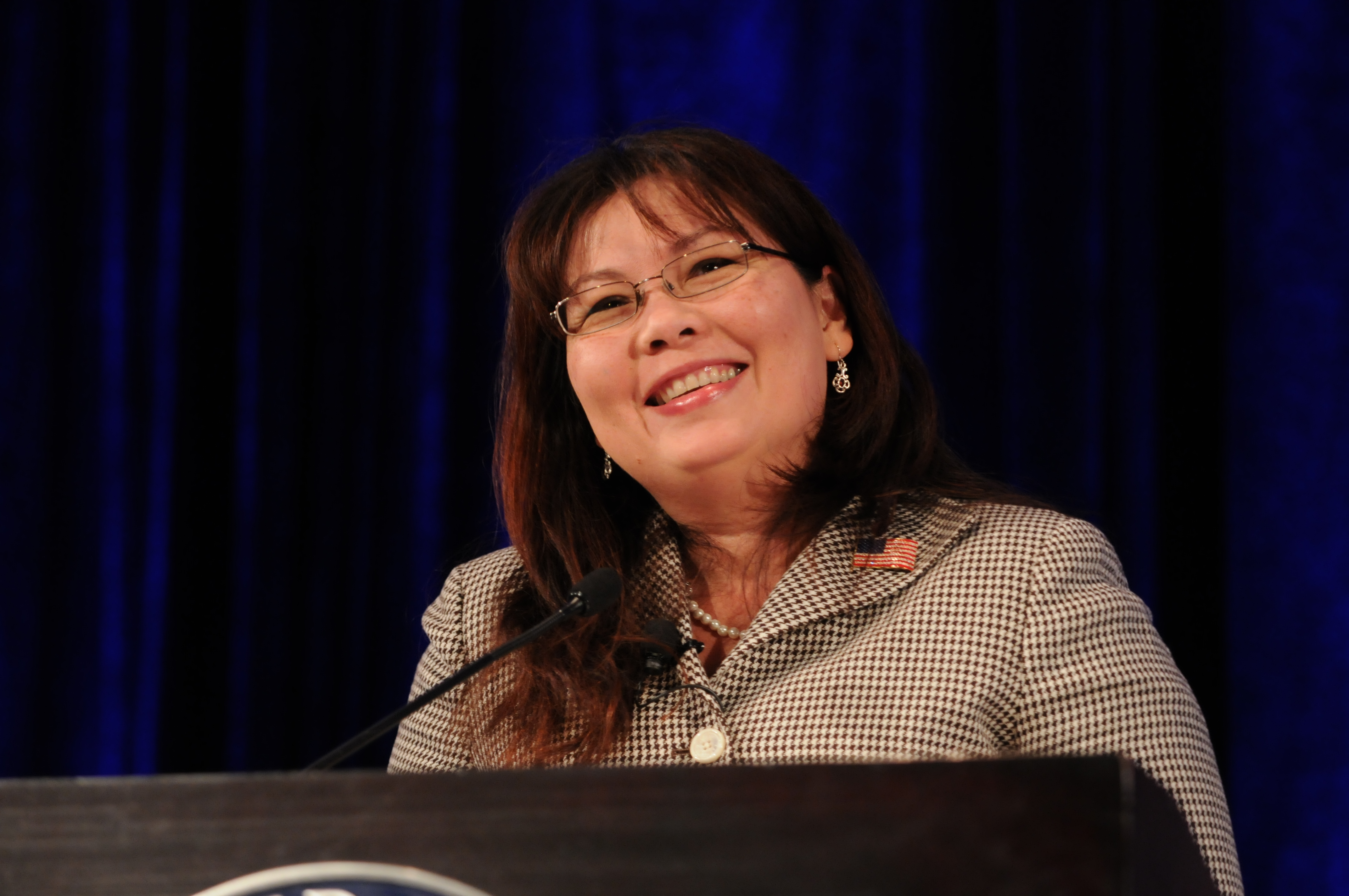In the image, a smiling woman stands behind a dark brown wooden podium, centrally positioned within the frame. Although the podium sports a partially visible logo, the focus is drawn to the woman at its center. She has brown hair with red highlights, styled straight with bangs and reaching past her shoulders. She wears square wire-rimmed glasses and a pearl necklace, complementing her thin black and white gingham jacket adorned with a pink ribbon on the collar and a United States flag pin on the lapel to her right. Her round face and prominent cheekbones are highlighted by her big smile, revealing her top row of teeth. In front of her, a thin stick microphone with a black fuzzy head is positioned, capturing her voice. The backdrop is dominated by a velvety blue curtain, suggesting an indoor setting appropriate for a presentation or speech. The colors in the image include shades of black, dark blue, brown, tan, pink, orange, and gray.